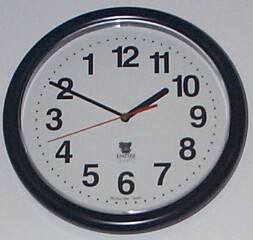This photograph features a white clock with a prominent black ring encircling its border. The clock appears to be designed in a reverse orientation, with its numbers arranged in descending order from 12 to 1, moving counterclockwise instead of the traditional clockwise direction. The current time displayed on the clock indicates 10:50 and 42 seconds, assuming the clock operates backwards; if it were running normally, it would display a time of 2:10 and 17 seconds. The clock's numerals are bold and black, contributing to its striking, unconventional appearance.